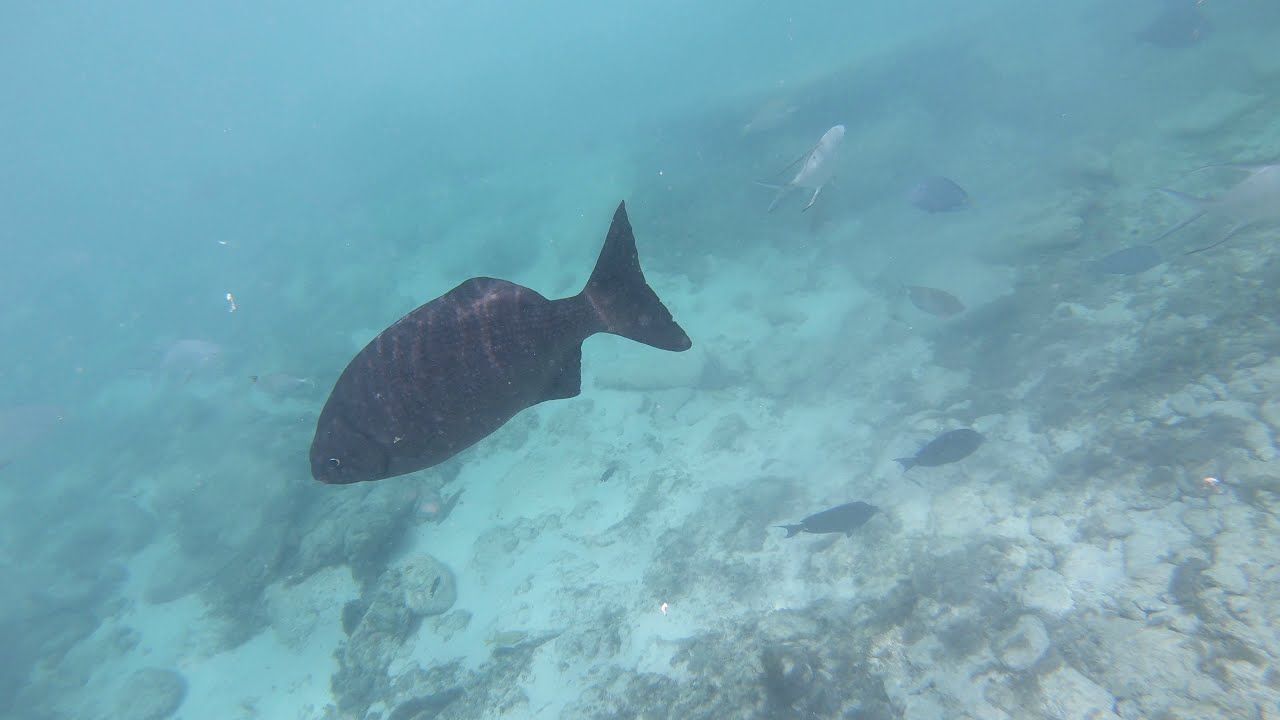This underwater scene captures a teal-colored ocean with clear, though slightly hazy, water. The main focus is a distinct fish starting about 60% up from the bottom and oriented towards the lower left-hand corner, roughly at the 7:30 to 8:00 position. This fish is predominantly black with lighter stripes, possibly deep purple or rose, although it's challenging to discern the exact hues due to the water’s bluish-green tint. The fish's tail is central to the composition, pointing upward, while its head angles downward. It also features brown and lighter brown stripes with a black-tipped fin.

Surrounding this fish, the scene includes a diverse array of smaller fish in the background. To the right, a white fish swims upwards towards the water’s surface. Additionally, scattered around are darker, almost black, fish that seem smaller due to their distance, creating a sense of depth. The ocean floor is comprised of a strikingly white sandy bottom overlaying dark gray rocks, adding textual contrast. Further adding to the scene are specks of reflective material, possibly bubbles or metallic particles, contributing to the scene's dynamic, underwater ambiance.